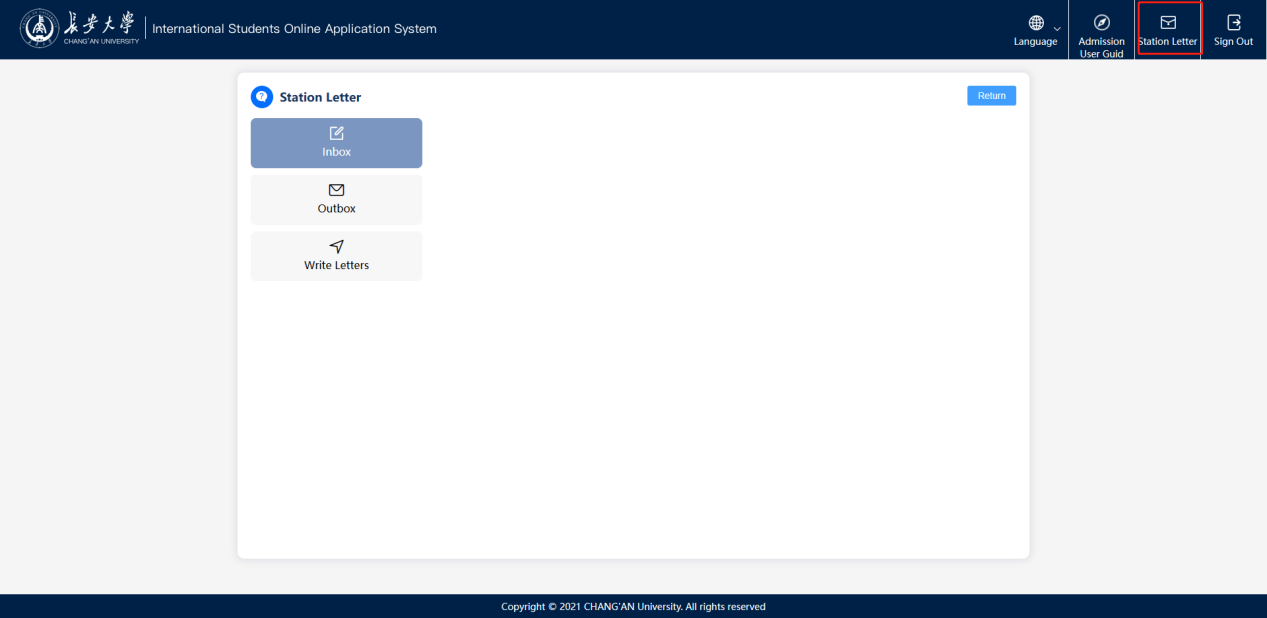The web page's interface is primarily white with prominent blue elements contributing to its clean and organized look. The top section features a bold blue header that spans the width of the page, adorned with white text. Starting from the left, the header begins with a series of easily recognizable icons followed by the text, "International Students Online Application System," clearly indicating the purpose of the page.

On the right side of this blue header, there are four distinct sections that provide drop-down menus or navigational options. The first section, labeled "Language," includes a drop-down arrow for selecting a preferred language. To its right, the "Admissions" section offers options related to the admission process. Next, the "Station Letter" segment likely pertains to communication and letter management. The final option, "Sign Out," features an exit icon for users to log out of the system.

In the main body of the screen, under the "Station Letter" section, users can navigate through three different selectable areas: "Inbox" for incoming messages, "Outbox" for sent messages, and "Write Letters" for composing new correspondence. 

At the bottom of the page, a slender, dark blue information bar runs across the screen. Centrally located within this bar, copyright information is clearly displayed, ensuring users are informed about the content ownership and usage rights. This detailed layout facilitates intuitive navigation and ensures ease of use for international students managing their applications online.